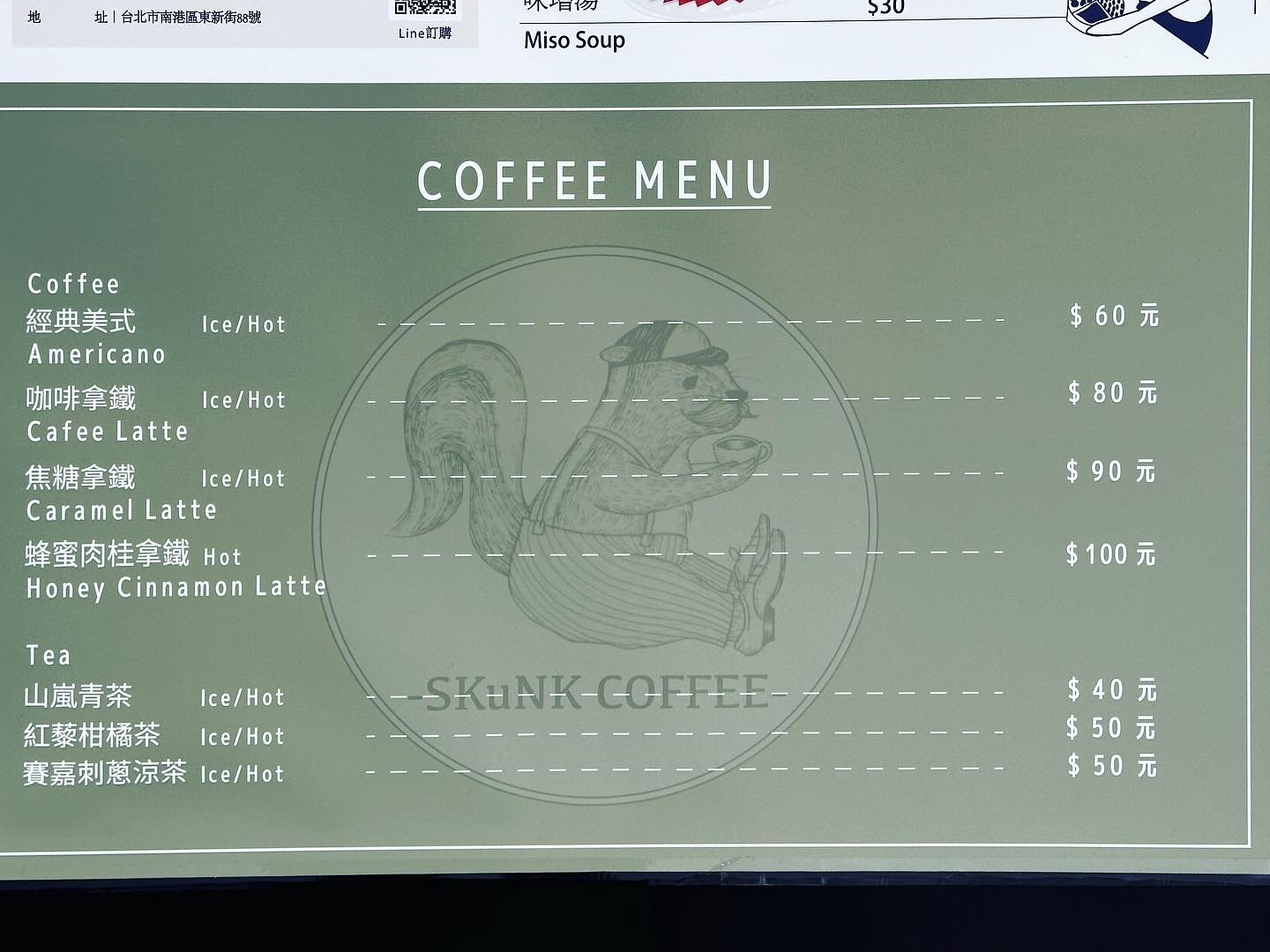A screenshot of a coffee menu from a website, prominently displayed against a green background. The top of the image shows part of a browser tab, indicating it is a digital capture. Below, the heading "COFFEE MENU" is centered in the middle of the page, with the letters spaced widely apart and underlined in white text.

On the left side of the menu, various beverage options are listed in both English and Mandarin/Cantonese. The options include:

- Coffee (Ice/Hot)
  - Americano
  - Café Latte
  - Caramel Latte
  - Honey Cinnamon Latte
  - Tea

Corresponding to these items on the right side of the menu are the prices, written in Chinese currency, though not specified as Yen. 

In the middle of the menu, there is a whimsical illustration of a skunk wearing a baseball cap, encircled, with the label "Skunk Coffee" beneath it.